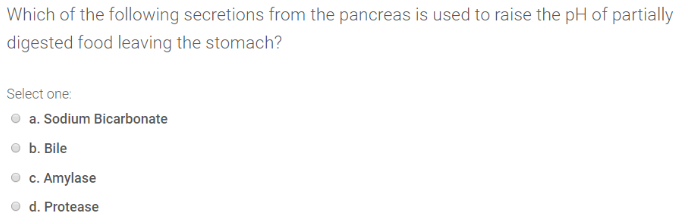This image is an educational screenshot comprising solely of text, with no photographic or illustrative elements. It features a multiple-choice question from an unidentified source. The question reads: "Which of the following secretions from the pancreas is used to raise the pH of partially digested food leaving the stomach? Select one." Four answer options are provided, each accompanied by a radio button: 
A) sodium bicarbonate, 
B) bile, 
C) amylase, 
D) protease. 
As depicted, none of the radio buttons have been selected by the user. The screenshot is in a landscape orientation, being wider than it is tall. The image contains no living organisms, people, or objects such as birds, animals, fish, lizards, snakes, plants, flowers, trees, buildings, bridges, automobiles, bicycles, or motorcycles.